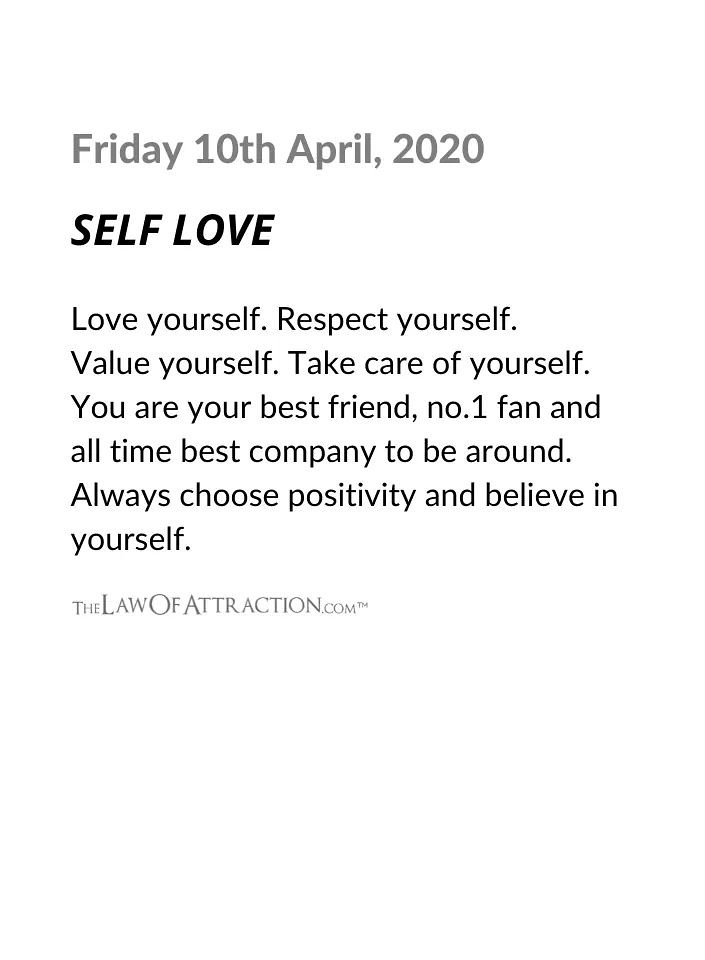The image consists of a plain white background with a motivational quote in different fonts and colors. At the top, in grayish lettering, it displays the date "Friday 10th April 2020." Below the date, in bold black letters, is the title "self-love." Following this, in smaller, non-bold black lettering, the quote reads: "Love yourself, respect yourself, value yourself, take care of yourself. You are your best friend, number one fan, and all-time best company to be around. Always choose positivity and believe in yourself." At the bottom of the image, in gray writing, is the source "thelawofattraction.com" accompanied by a trademark symbol. The image is simple with no additional designs, solely focused on delivering a clear and inspiring message about self-love.